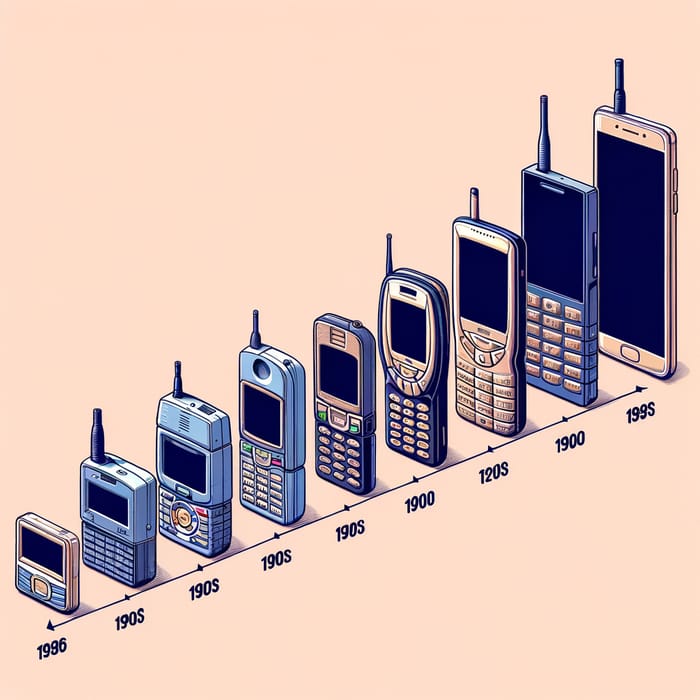This detailed infograph illustration, set against a salmon pink background, depicts the evolution of cell phones over time. Arranged diagonally from the bottom left to the upper right, the timeline begins in 1996 and progresses through a series of model numbers rather than specific dates, generally marked as "190S" and "199S." The sequence starts with a small, basic paging device in the bottom left corner and grows increasingly advanced in size and complexity, culminating in an iPhone at the top right.

Each cell phone in the lineup features a distinctive antenna except for a few, including the final smartphone, making the presence of antennas a notable characteristic. Most phones have physical buttons typical of late 1990s to early 2000s designs. The color palette includes navy blue and light blue phones contrasted against the consistent salmon background. The graphic effectively highlights the technological advancements and design changes of cell phones over the years.